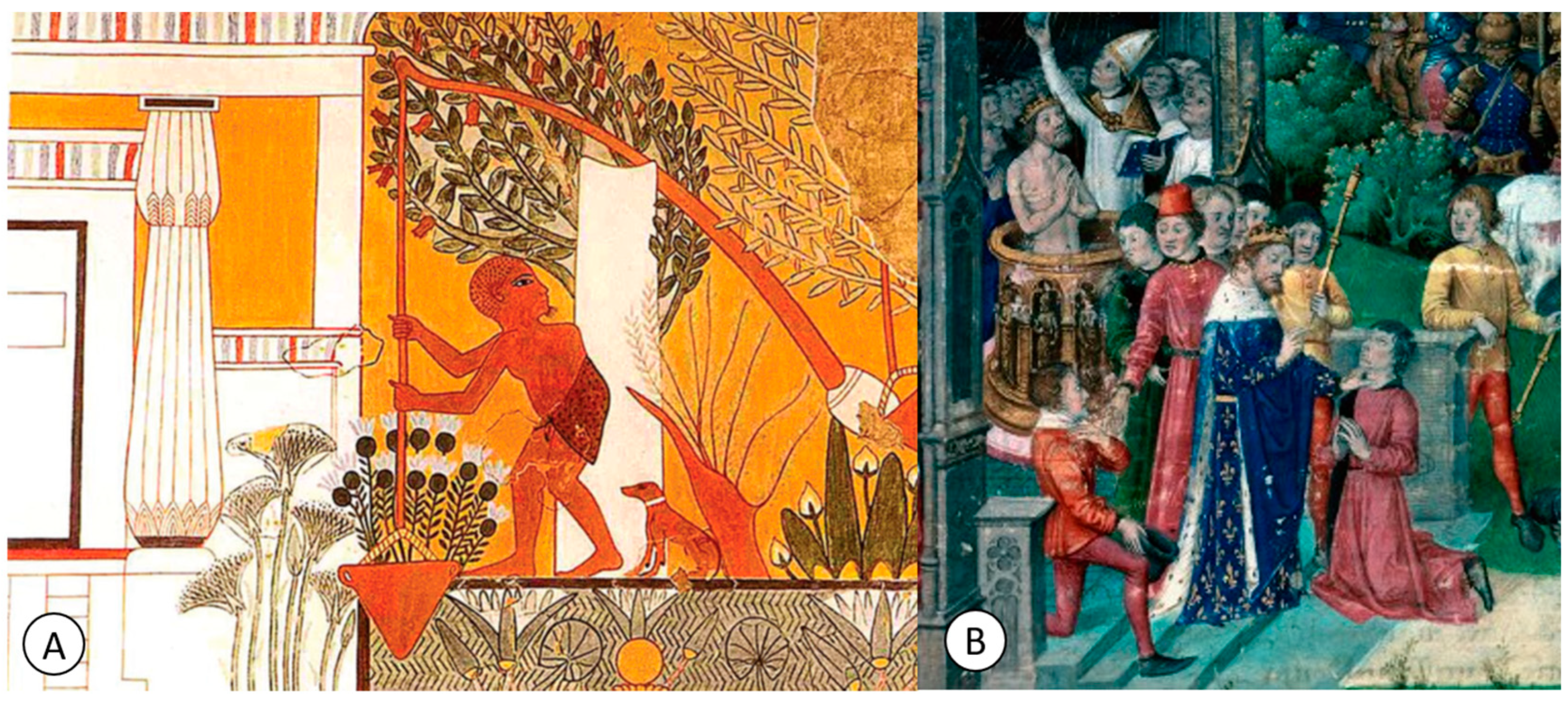The horizontally oriented image is divided into two distinct sections, each showcasing a different style of art. The left side, which occupies roughly 60% of the canvas, features an Egyptian-themed artwork labeled 'A' in a black circle with a white interior. This image depicts a bald, orange-toned figure wearing a simple brown garment around his waist, who appears to be gardening or performing some task with a device planted in the ground. Beside him is a small orange dog, with leafy trees and white columnar structures completing the scene, set against a bold, colorful backdrop of deep greens, browns, oranges, and reds.

On the right side, taking up the remaining 40%, is a medieval Renaissance-style painting labeled 'B' in a white circle with a black outline. This piece is dominated by hues of blues, reds, and greens and depicts a crowned figure in a rich blue robe, likely a king, surrounded by a mix of standing and kneeling figures wearing various colored garments. The scene appears to portray a significant ceremonial or religious moment, possibly an anointing, against a green backdrop with hints of foliage and a darker overall ambiance.